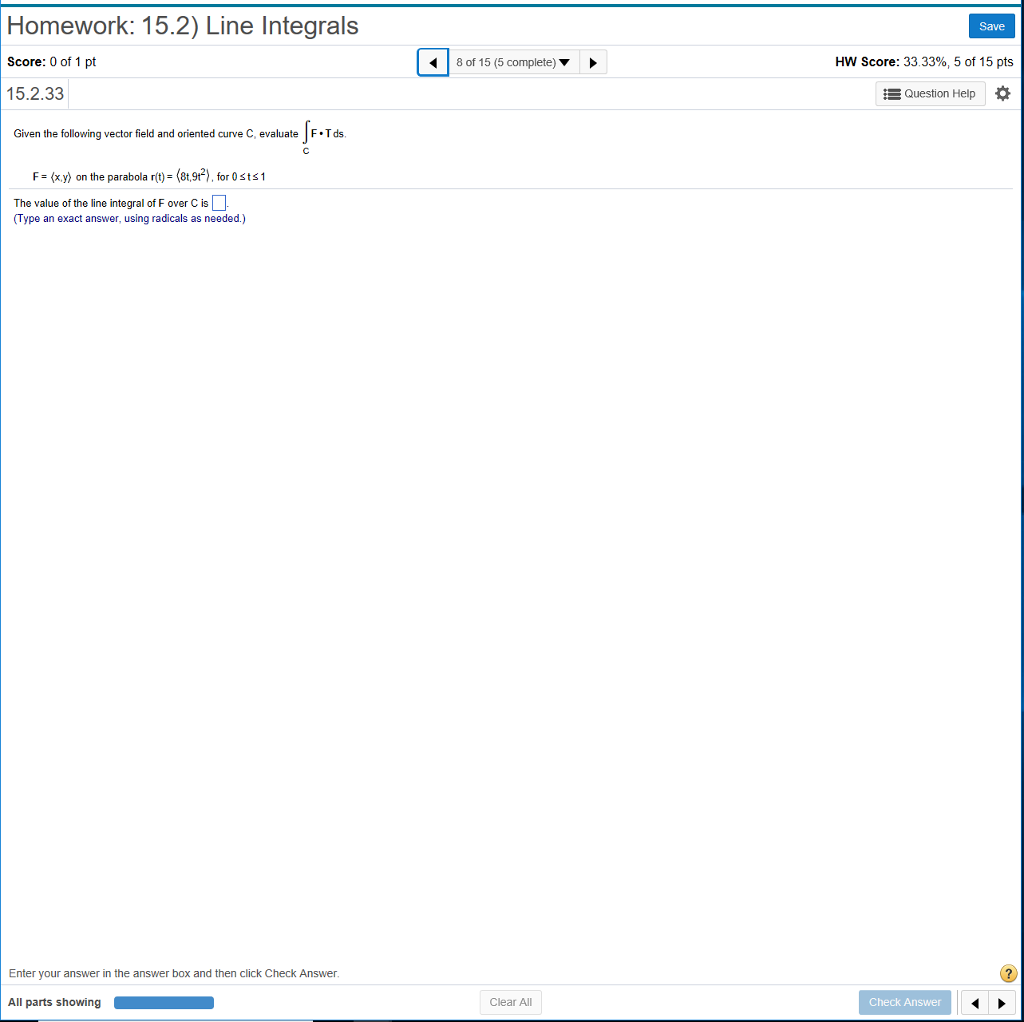This image features a white background predominantly filled with black text. In the upper left-hand corner, the word "Homework" is displayed, followed by "15.2 (Line Integrals)". To the right, there is a blue "Save" button situated in the far-right corner. Directly below "Homework," the text shows "Score: 0 of 1 point". Adjacent to this, there are navigation icons including a back arrow, a forward arrow, and a dropdown menu displaying "0 of 15 (5 complete)", with a blue square highlighting the back arrow. Further to the right, it indicates "HW Score: 33.33% (5 of 15 points)".

Below this section, the text reads "15.233" with a checkbox next to it, along with a "Question Help" button and a gear icon positioned to the far right. The content below poses a question, stating "Give the following vector field an oriented curve C, evaluate F + F_cl of C". The lower portion of the image depicts a user's attempt to solve the question. The bottom half of the image remains mostly white, except for a "Check Answer" button located at the bottom right.